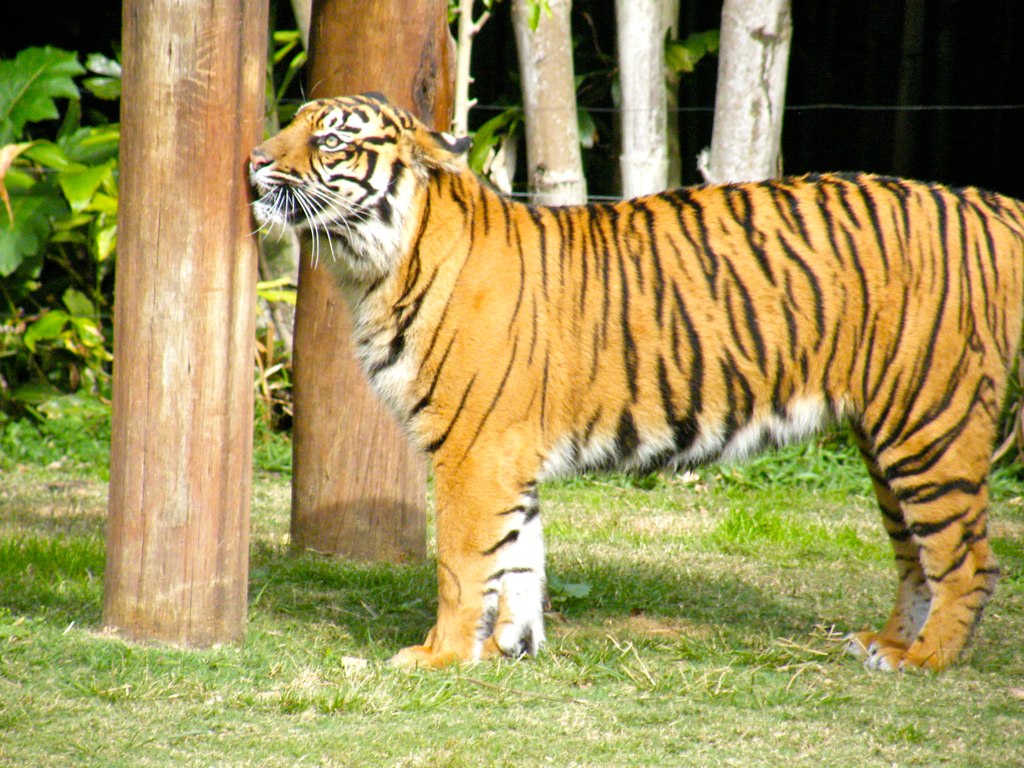The photograph captures a large, adult tiger with vibrant orange fur accented by black stripes and a white underside, including its belly, chest, and the area around its mouth and eyes. The tiger's face features white whiskers and striking yellow eyes with small black irises. It stands in a sunny, flat grassy area, rubbing its face against one of two smooth wooden logs. The background reveals the tiger's captivity, with a wire fence enclosing the area. Behind the fence, there are light brown tree trunks, various green vegetation, and bushes, creating a mix of natural and constructed habitats. The setting is reminiscent of a zoo or sanctuary, with short grass and visible tiger shadows indicating bright daylight.